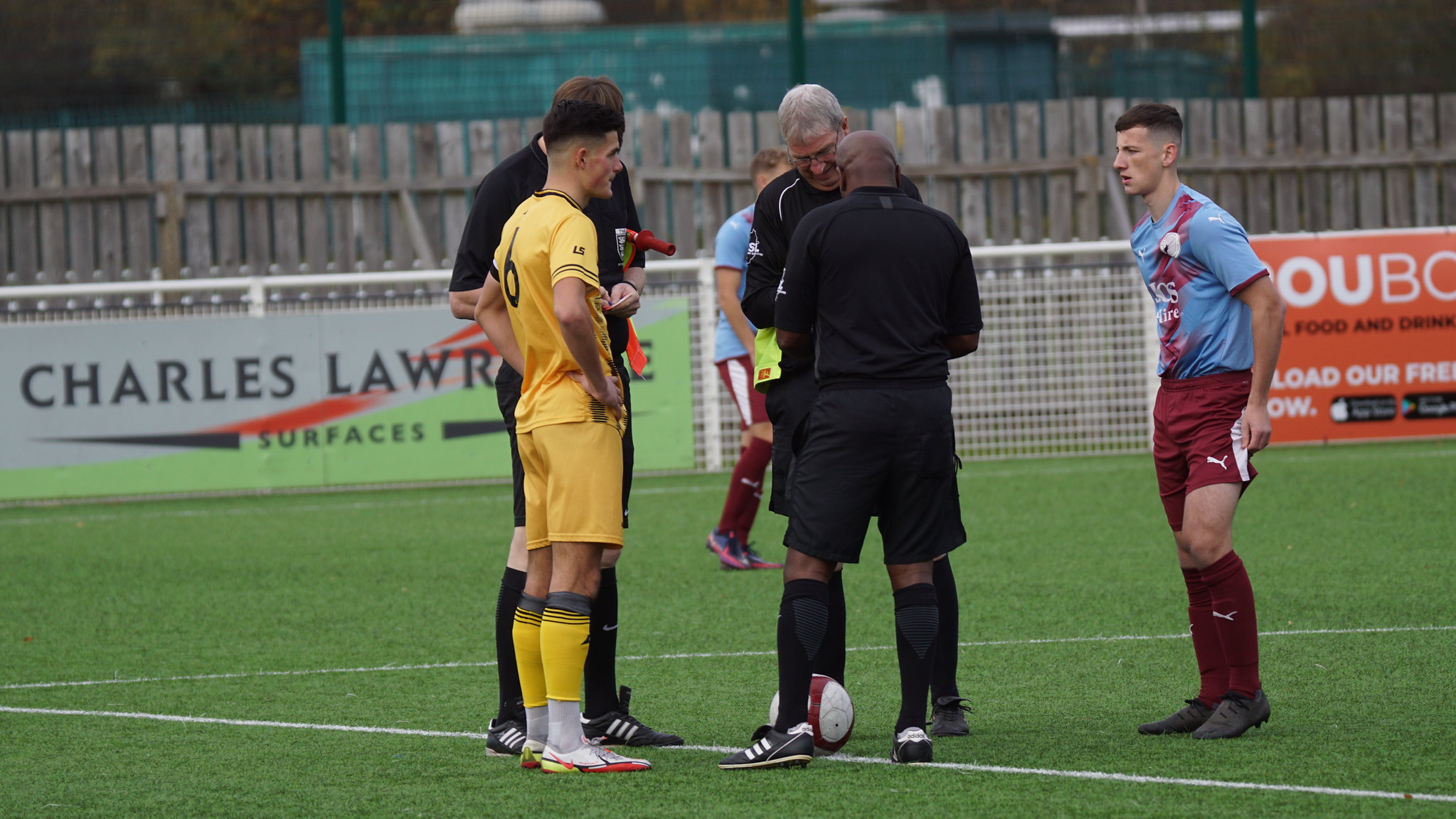The image captures a scene on a soccer field, likely during a game or pre-game meeting. Six men are present on the green artificial turf. At the center are two referees in black uniforms, one with his back to the camera, standing next to a soccer ball at his left foot. He appears to be talking to another referee with silver hair, whose face is partially visible. To the right of the referees stands a younger player with short hair, sporting a blue and maroon uniform—maroon shorts and socks paired with a blue shirt. On the left side of the referees, another player is dressed in an all-yellow uniform, including yellow socks. Adjacent to him, there's a man in black whose face isn't visible. 

In the background, a wooden plank fence and a taller green metal fence partly obscure some advertising signs. One billboard clearly reads "Charles Lawrence Surfaces," while another is orange and partially legible with the text "OUBO" visible. The goal net lies further back behind the fences, adding to the sense of a professional or semi-professional soccer setting. The scene, enriched with vibrant colors like black, white, yellow, maroon, blue, orange, red, brown, and green, suggests a lively encounter on the field.